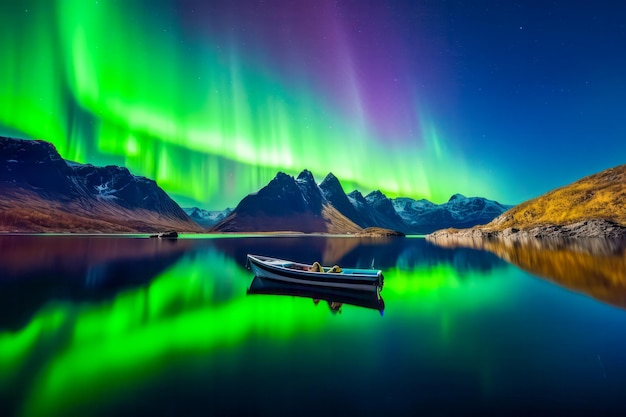The image, possibly an artistic creation, captures a breathtaking scene with a serene boat positioned in the center of a tranquil lake. In the foreground, the lake's still, dark blue water reflects vivid shades of lime green from the Northern Lights above. The lights, primarily lime green with hints of purple at the top, stretch across the sky in vivid, dynamic streaks. The backdrop features majestic snow-covered mountains, their white peaks illuminated by the ethereal glow. To the right, grass-covered hills add a touch of earthy green, contrasting with the snowy summits. The image’s left portion shows the lake extending between two land sections, enhancing the depth of the scene. Despite the subtle reflections of the brown mountains, the Northern Lights' neon brilliance dominates both the sky and the lake's mirror-like surface, creating a harmonious blend of celestial and terrestrial beauty.